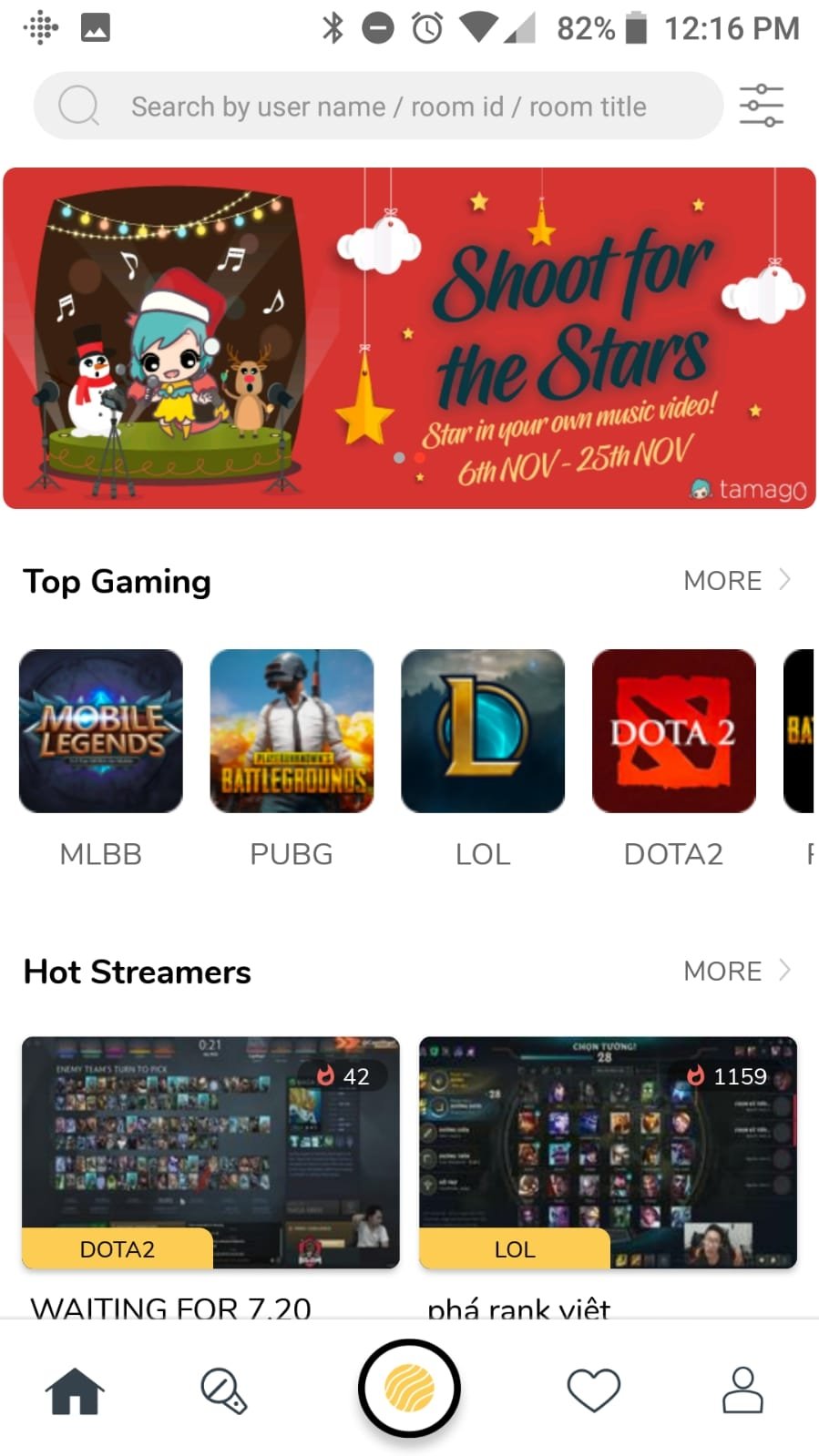**Caption:**

The image is a screenshot of the second page of an app. At the top, there is a gray search bar with the placeholder text "Search by username / room ID / room title." Above it, a red banner on the right displays the slogan "Shoot for the stars." On the left side of the screen, there's an illustration resembling a small stage featuring various comic characters: a snowman, a girl with green hair wearing a Santa hat, and a reindeer. The stage is adorned with hanging cloud and star ornaments. The text "Star in your own music video: 6th November through 25th November" is prominently displayed below the illustration.

Underneath this section, there’s a heading titled "Top Gaming" on the left and a "More" option on the right, accompanied by a forward arrow icon. Below this, four game thumbnails are displayed with their respective titles: Mobile Legends, PlayerUnknown's Battlegrounds, League of Legends, and Dota 2.